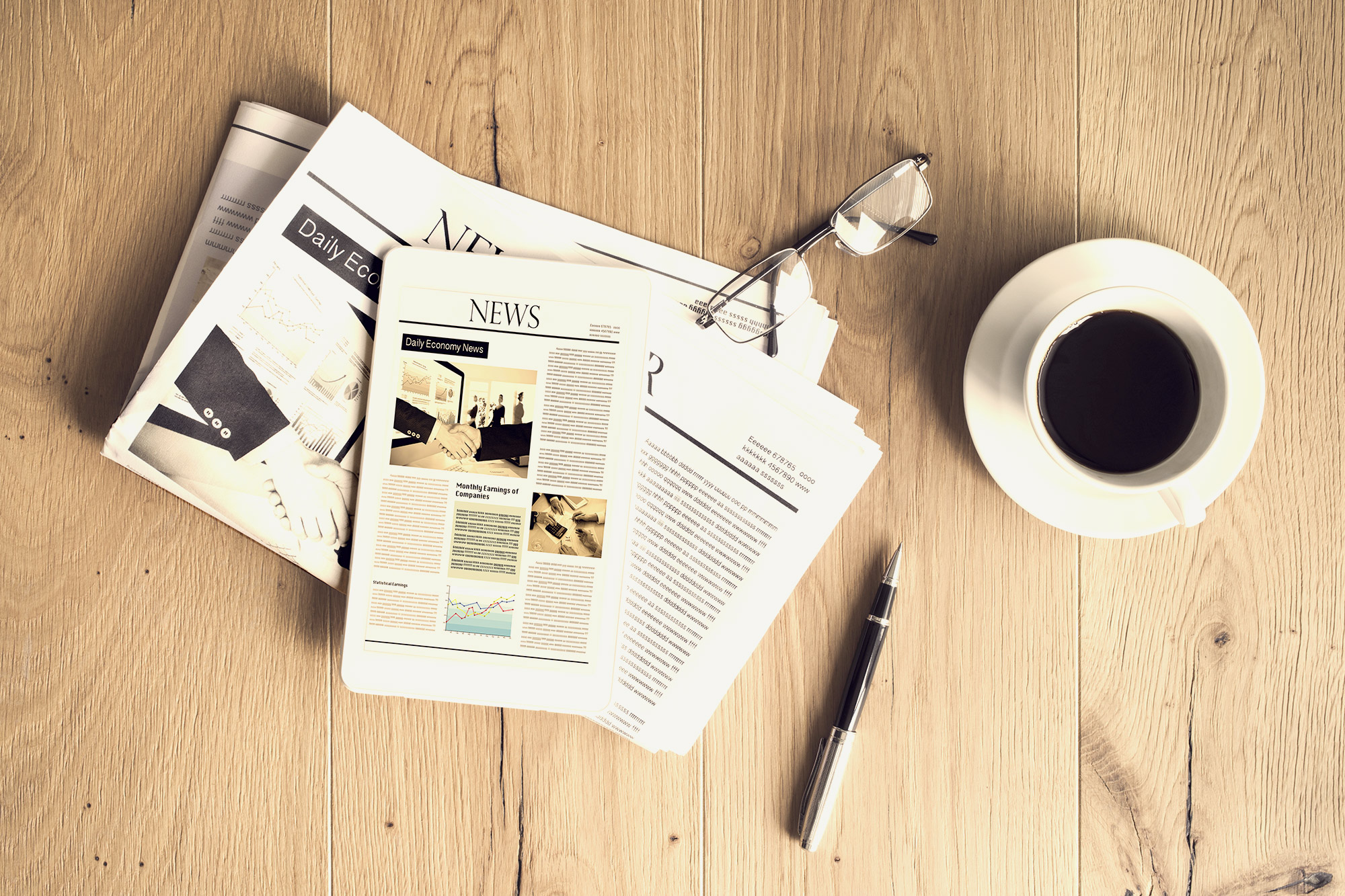The image showcases a rustic, light beige wooden table composed of various unpolished panels, revealing natural patterns and cracks. At the center is a white ceramic cup filled with brown liquid, presumably coffee, resting on a matching white circular plate. Next to the cup lies a high-end black ballpoint pen with a silver back and tip. Spread across the table is a newspaper, prominently displaying the word "NEWS" in all capital letters, and what appears to be a newsletter, both featuring dummy text and random characters. Above the newspaper sits a pair of glasses. The image is bathed in natural sunlight, casting a warm glow on the coffee cup and the newspaper, enhancing the rustic feel of the wooden tabletop.